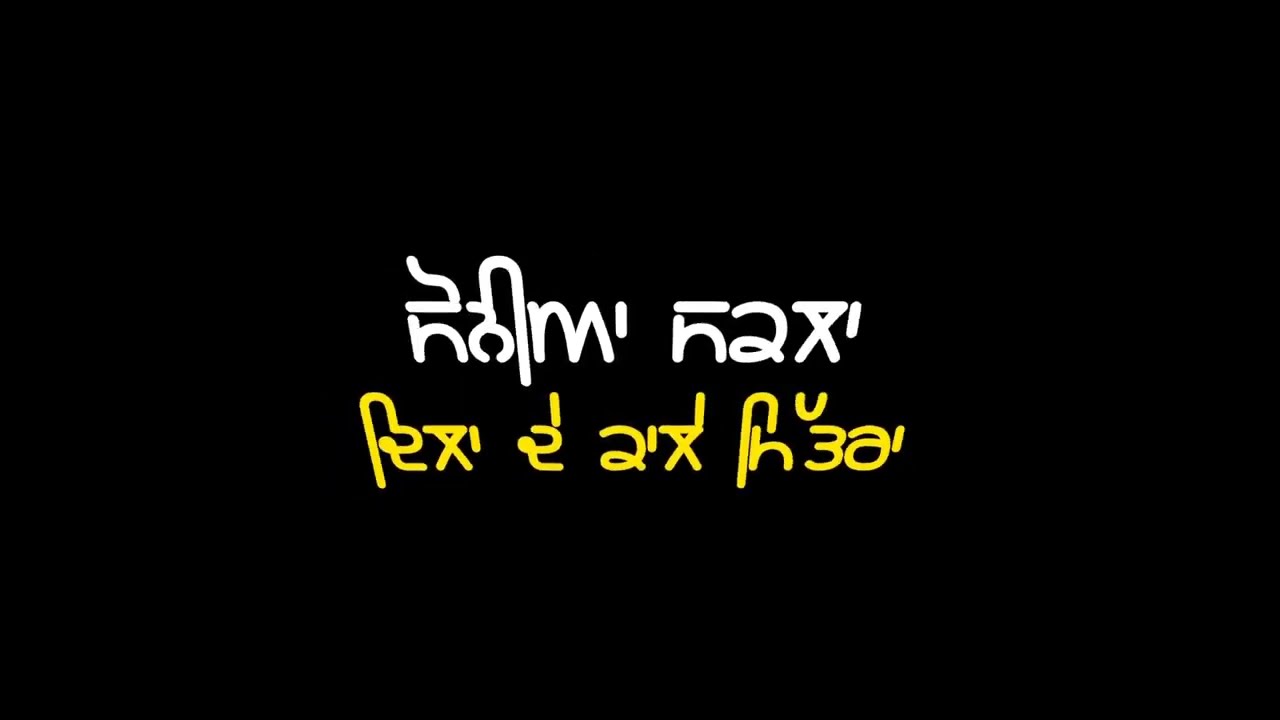The image is rectangular, with dimensions approximately six inches wide and four inches tall, featuring a simple and stark design. The background is entirely black. Centrally placed, the image contains two rows of text, each in a different color and written in an unfamiliar, possibly symbolic script. The top row contains two words in white text, while the bottom row has four words in yellow (described as gold) text.

Specifically, the top row's first symbol resembles a lowercase 'n' with another 'n' above it, rotated 90 degrees counterclockwise. Following this is a symbol vaguely like a 'C' facing downwards, with a curve extending from its top, and a long 'U' shape stretching down to the right. Next, there appears to be an 'M' with an adjacent short apostrophe. The second word of the white text starts with a character similar to an 'n' with a long dash over it, followed by what looks like the number '2', and then an 'X' with a horizontal dash over it, ending with an apostrophe.

The bottom row's first symbol in yellow text starts with a form reminiscent of the top part of an 'F', transitioning into a shape like an 'L', and then down into a 'K', followed by an 'X' with a bar over it, and an apostrophe. The next symbol resembles an interaction between a number '2' and a lowercase 'e', topped with a horizontal dash. The third word starts with a character resembling the number '2', followed by an apostrophe, then an 'X' with an 'L' resting on it. The final word includes a long shape similar to a candy cane hovering over a lowercase 'h', partnered with the number '3'. Near the '3' is a small 'U' to the left and the beginning of a lowercase 'a' with an apostrophe on the right.

Overall, this highly detailed image features text in an unknown language, with precise and peculiar symbolic representations.